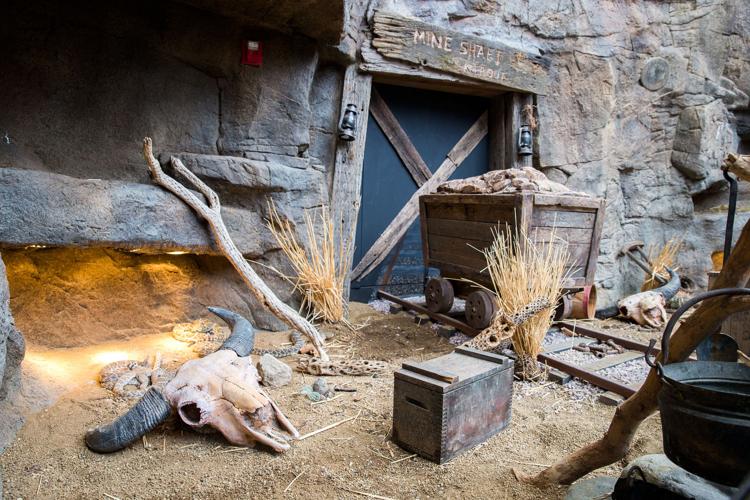The image captures the front facade of a meticulously recreated old Western mine, likely part of a museum exhibit. The mine entrance, integrated into a rocky mountainside, features a wooden frame topped with a plaque that reads "Mine Shaft." Flanking the entrance are two lanterns, while two wooden planks form an X across the closed doorway. A set of metal rails leads up to the entrance, where an old mine cart filled with rocks rests. Scattered around the mine entrance are artifacts that enhance the historical ambiance: a wooden box, worn cooking pots, large branches resembling walking sticks, and several cow or bull skulls. Embedded lights beneath some stones cast an ethereal glow, illuminating the scene and adding to the staged, yet authentic feel of the exhibit.